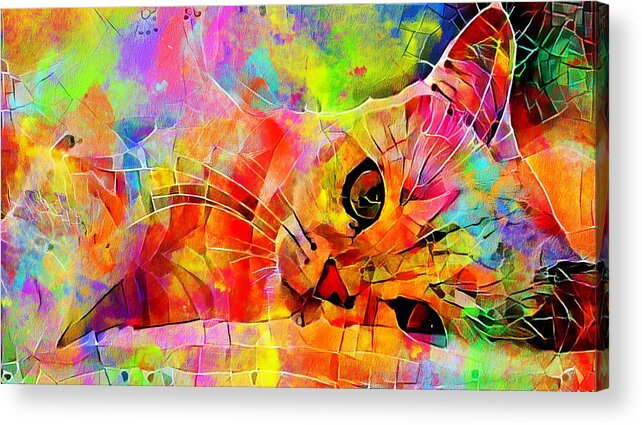This abstract painting vividly captures a cat lying on its left side, with its head resting on its left cheek on the right side of the composition. The cat's form is constructed from an array of geometric shapes, including squares, rectangles, and curved lines, evoking a mosaic-like appearance. The artwork is alive with bright and contrasting colors, such as lime green, pink, fuchsia, yellow, red, and fluorescent green, blending and splattering to enrich the visual experience. The cat's features are intricately detailed, with its prominent eye showcasing multiple colors and outlined in black. Despite the stylized, fragmented depiction, the cat gazes straight ahead, creating a captivating focal point. Overall, the interplay of geometric patterns and bold colors enhances the abstract aesthetic, making the painting a striking and dynamic representation of a reclining cat.